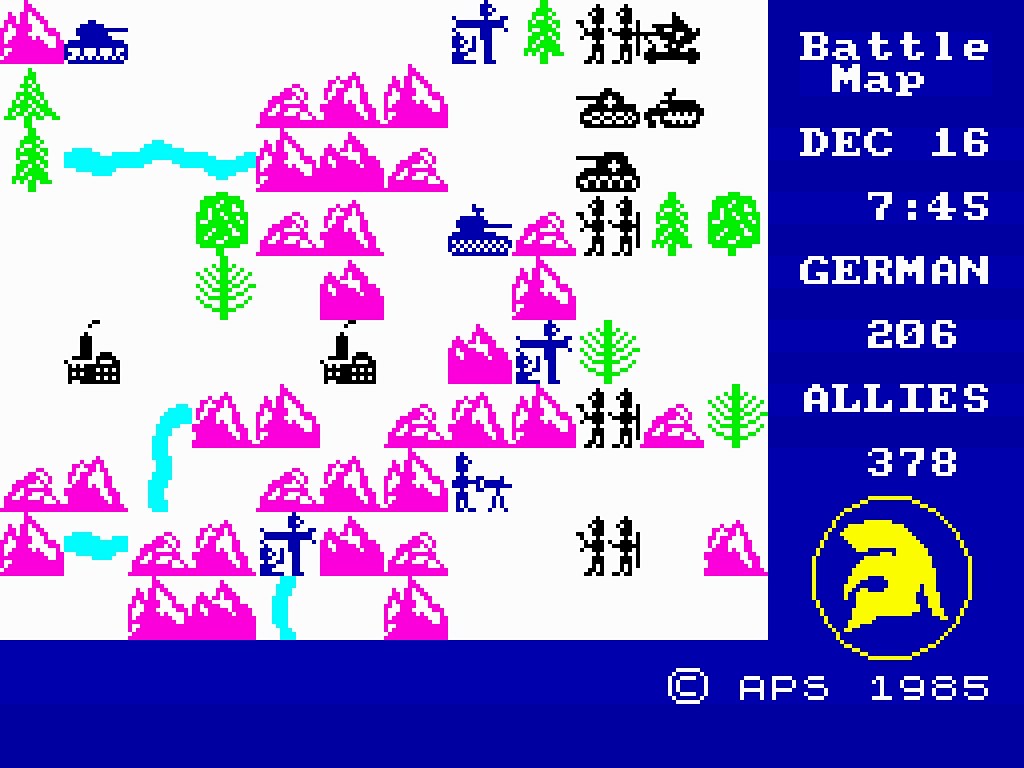The image is a screenshot from an old, pixelated video game called "BattleMap," which features graphics reminiscent of the Atari era, dated December 16th, 1985. Dominating the scene is a large, white diagonal expanse that runs from the upper left corner down about three-quarters of the way through the page, stretching two-thirds across to the right. Surrounding this area are numerous purple mountains or hills, interspersed with scattered green trees.

The game displays several military elements: blue tanks oriented rightward are positioned across the map, with one in the center and another in the upper left. Sporadically placed are also black tanks facing left. Among these are four blue soldiers and several black soldiers, all directed towards the right. On the second row from the right, the black soldiers are aligned in a sequence starting with two at the top, then two tanks, followed by another pair of black soldiers, a leaf, and finally, four more black soldiers in two pairs.

In addition to the soldiers and tanks, there are two black industrial buildings with smokestacks emitting smoke, one notably appearing in the middle of the map.

The right side of the image features text in white, stating "Battle Map" at the top, followed by "December 16th," "745," "German 206," and "Allies 378." Below this text is a yellow circle containing a stylized, sideways 'M' symbol, which resembles a battle sigil, and the letters "APS 1985" in white beneath the circle. The graphics overall are simple and low-resolution, typical of DOS games from the mid-1980s, with elements rendered in basic dots and lines.